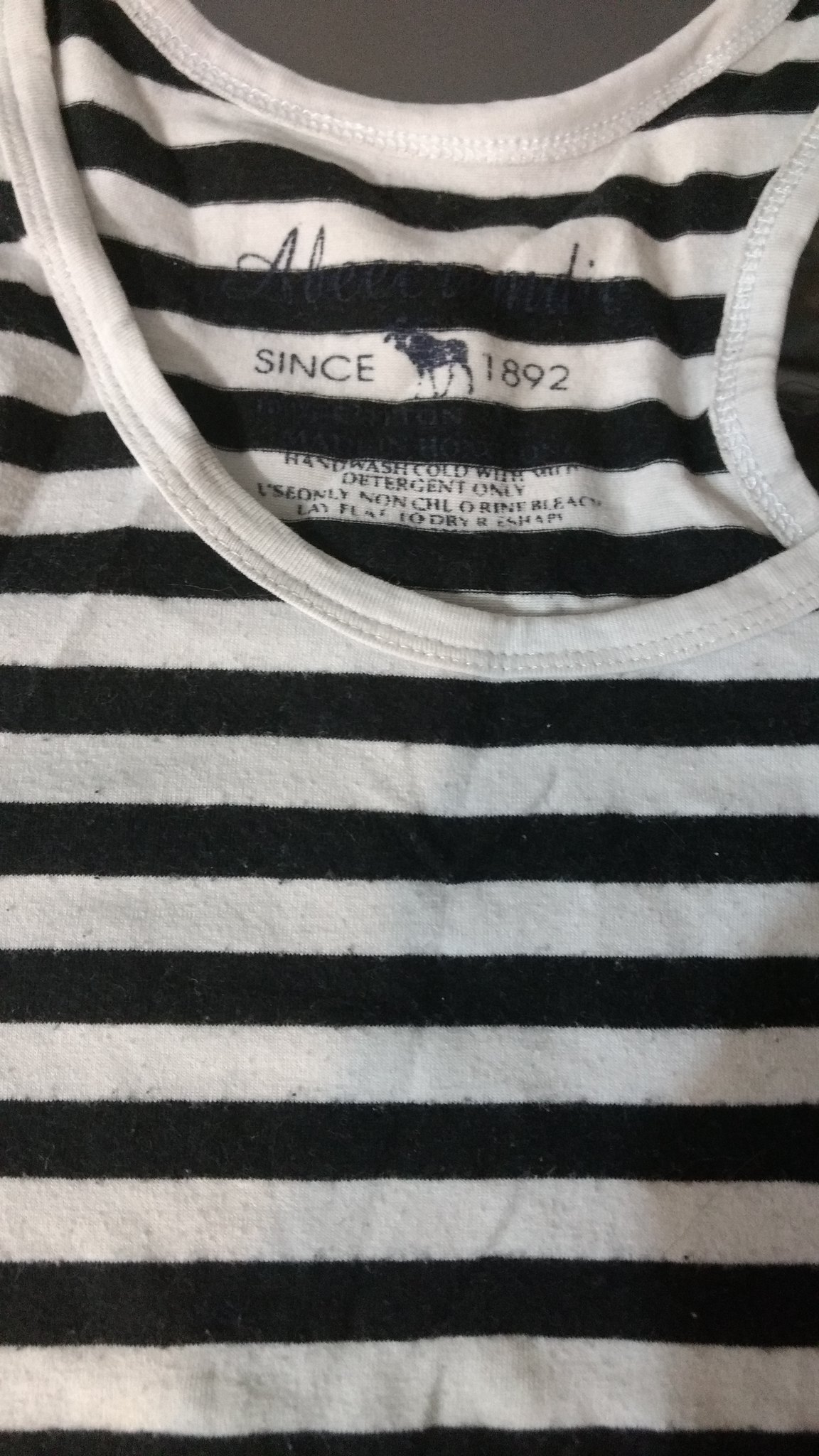The image features a stylish tank top with a predominantly white collar. The rest of the shirt showcases an alternating black and white striped pattern, running vertically from the top to the bottom. This striking pattern creates a bold visual effect. The bottom right portion of the shirt is mostly shaded, contrasting with the upper section, which is brightly lit.

In addition to the visual details, there is text incorporated into the design of the shirt. At the top, the text reads "Since 1892," accompanied by an illustrative symbol that seems to be a horse. Below this, there are care instructions that specify "hand-washed, cold, detergent-only, using a non-specified method." The collar also features meticulous white stitching along its edges, adding a polished finish to the garment.

The overall appearance of the tank top is both eye-catching and sophisticated, with careful attention to detail in both its design and construction.